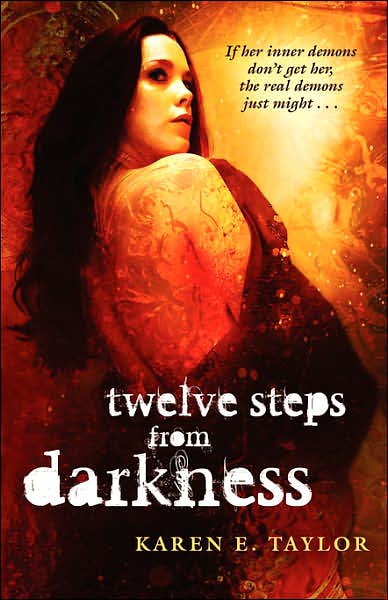The book cover for "12 Steps from Darkness" by Karen E. Taylor features a young woman in a side view pose, dressed in a dark red garment that is pulled down slightly in the front, revealing intricate tattoos and possible scarring on her exposed back and shoulders. Her long, dark hair cascades past her shoulders as she tilts her head back, glancing over her right shoulder towards the upper right corner. The background is a blend of red and yellow colors, resembling flames or a fire, creating a dramatic and intense atmosphere. Superimposed at the bottom in white typewriter-style text, somewhat smudged, are the words "12 steps from darkness," with "Karen E. Taylor" in all caps and a cream color beneath it. In the upper right-hand corner, in black italic type, the foreboding phrase reads: "if her inner demons don't get her, the real demons just might..." This compelling combination of photography, illustration, and graphic design suggests a story filled with inner and outer battles, enhanced by a tone of suspense and mystery.